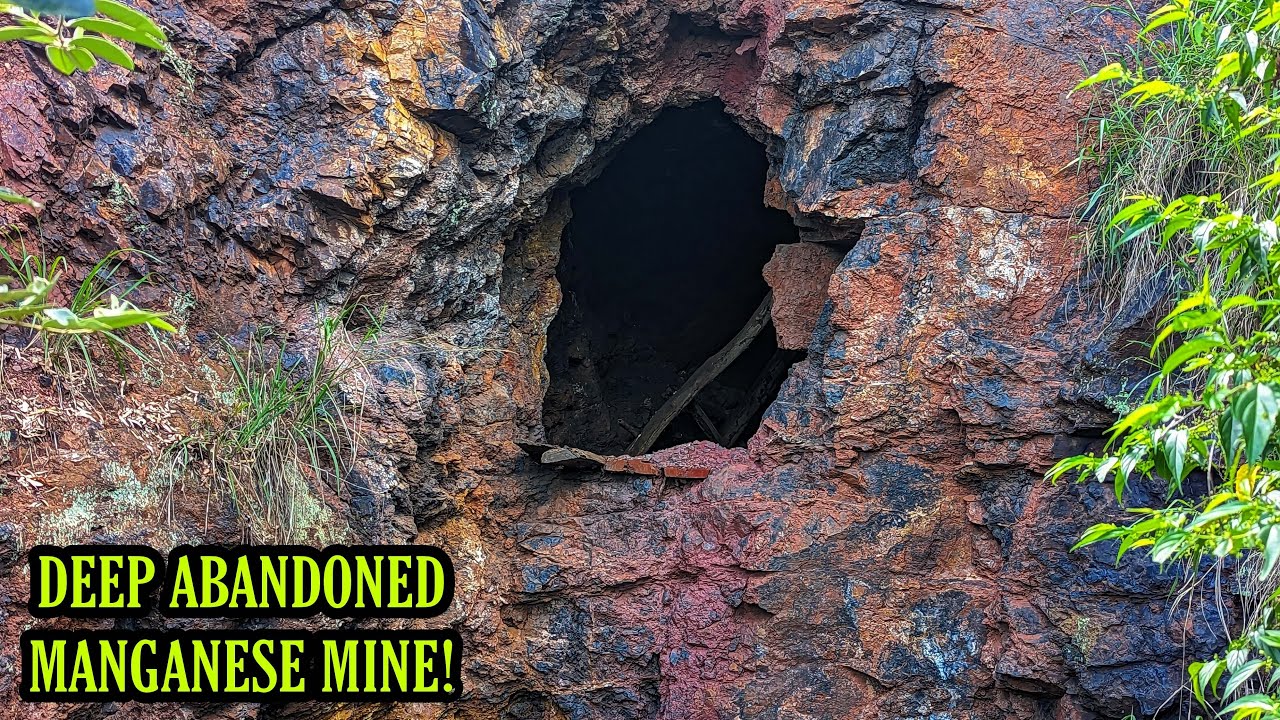The image showcases the entrance to a cave-like mine, identified by the bold text in the bottom left corner as "Deep Abandoned Manganese Mine," rendered in bright green and yellow fonts with a black outline. The entrance is roughly human-sized, leading into a foreboding dark void. The surrounding rocky cliff is a striking mix of deep rusty reds, oranges, dark blues, greys, and blacks, giving the impression of heavily rusted rocks. Sparse foliage is present, with small green leaves and blades of grass on both sides of the entrance, denser on the right. A piece of wood, possibly remnants of a ladder, is visible near the entrance, hinting at the mine's abandonment. The landscape appears rugged with no clear path or steps to the mine's entrance, reinforcing the wild and untouched nature of the site.